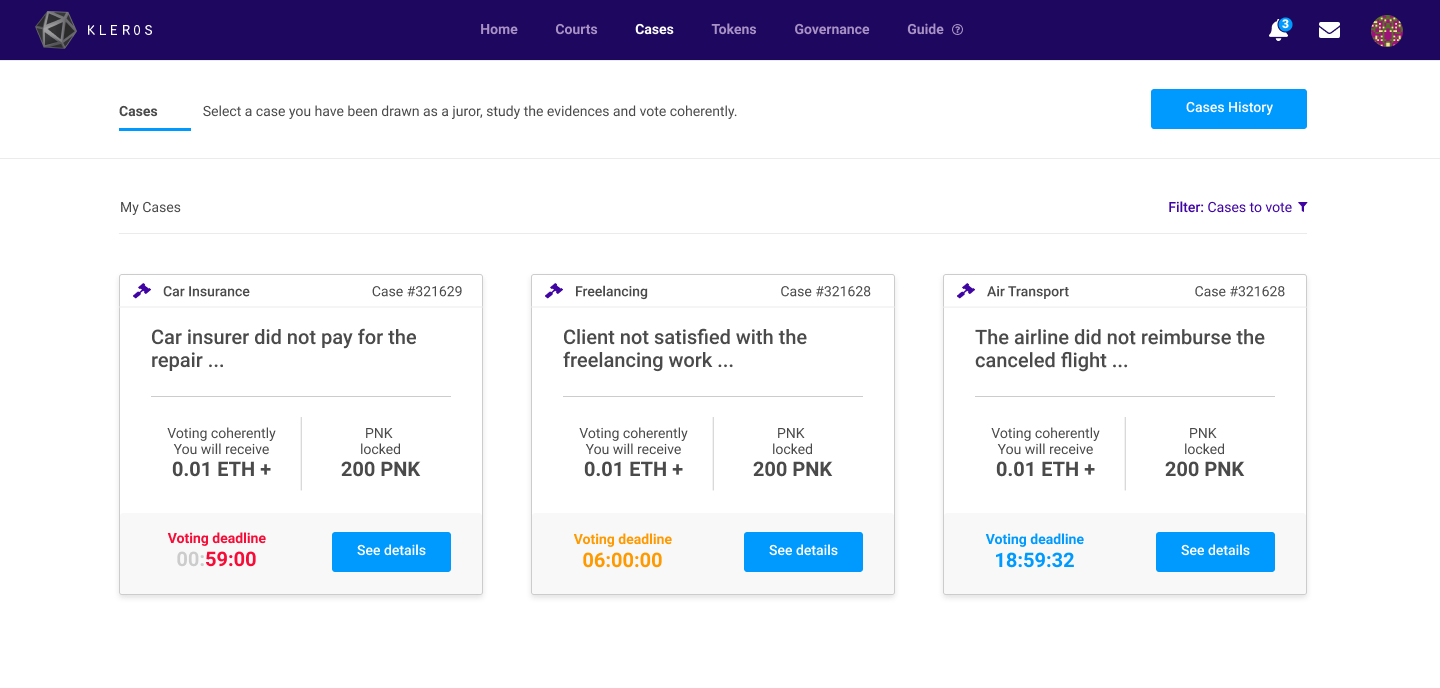A screenshot of the Kleros website, marked by a distinct purple border at the top. The header features the platform’s name, "Kleros," styled in bold next to a black hexahedron-shaped dice logo. Adjacent to this branding, the navigation bar includes options labeled "Home," "Courts," "Cases," "Tokens," "Governance," and "Guides." On the right side of the header, there is a bell icon with a notification count of 3, alongside mail and profile icons.

Below the header, the main content is focused on "Cases." It instructs users to select a case in which they have been assigned as a juror, undertake a detailed study of the presented evidence, and submit a well-reasoned vote. Several tabs are outlined for further navigation: "Cases History," "My Case," "Filter," and "Cases to Vote."

Three specific cases are highlighted:

1. "Car Insurance, Case 321629":
   - Dispute: Car insurer did not pay for the repair.
   - Incentive: Voting coherently awards you 0.01 ETH.
   - Requirement: 200 PNK tokens are locked.
   - Action: See details for more information.
   - Voting Status: In-progress.

2. "Freelancing, Case 321628":
   - Dispute: Client is unsatisfied with the freelancing work provided.
   - Incentive: Voting coherently awards you 0.01 ETH.
   - Requirement: 200 PNK tokens are locked.
   - Deadline: 6 hours remaining.
   - Action: See details for more information.
   
3. "Airline Reimbursement, Case 321627":
   - Dispute: Airline did not reimburse for the canceled flight.
   - Incentive: Voting coherently awards you 0.01 ETH.
   - Requirement: 200 PNK tokens are locked.
   - Deadline: 1859.32 remaining.
   - Action: See details for more information.